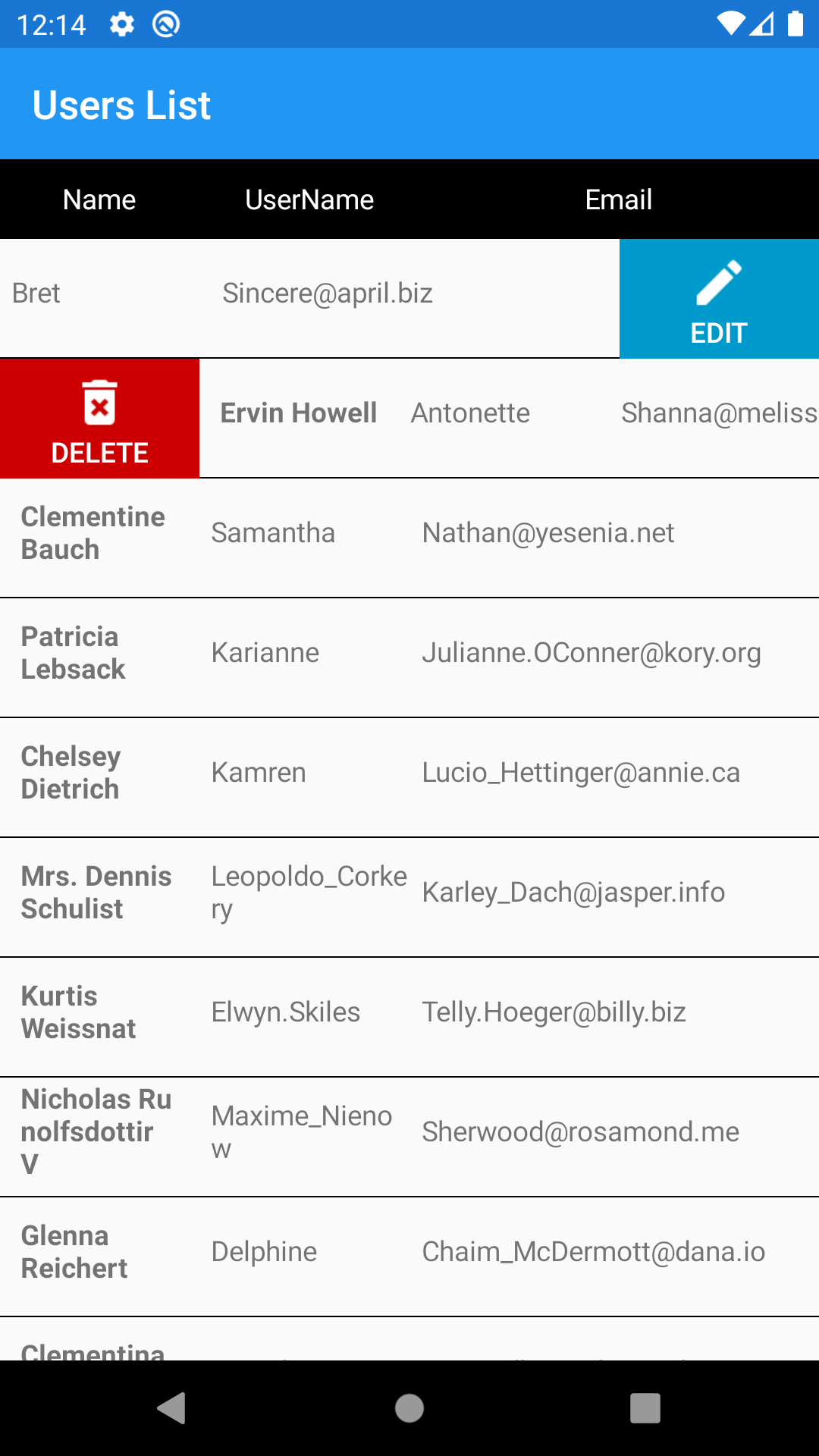In this screenshot, we see a user's list displayed on a mobile phone screen. At the very top of the screen, the time is shown as 12:14 PM. To the right of the time, there are a couple of status symbols, including a white Wi-Fi icon and a white battery icon, indicating the device's connectivity and battery status.

The background at the top of the photo is dark blue, transitioning to a lighter blue ribbon that spans across the top section. On the left side of this ribbon, the text "Users List" is displayed in white. Below this ribbon, there is a black bar that serves as a header for a table with three columns labeled "Name," "Username," and "Email."

Underneath these headers, multiple rows of user information are presented against a white background. The text within these rows is small and black. In the first row, the name "Brett Sincere" is listed, with "sincere_at_april" as the username, but the email field is obscured by a blue "Edit" button. The row below includes a red "Delete" button on the left, displaying the name "Irvin How," with the username "Antoinette" and an email beginning with "shannon@melissa..." which is cut off at the right edge of the screen. 

The overall layout is structured and captures a snapshot of a user's list interface from a mobile application.